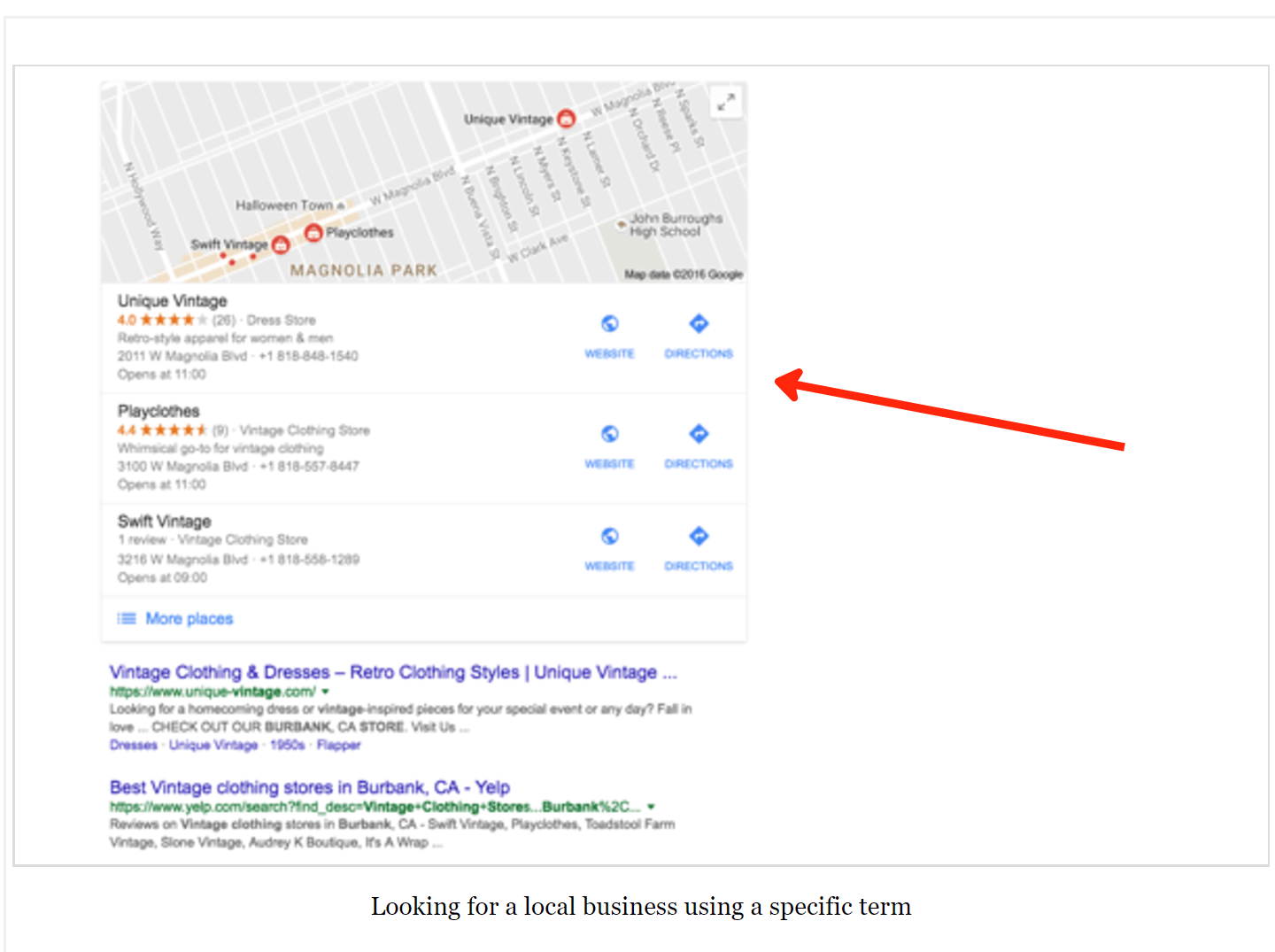**Caption:**

The image showcases a computer screen displaying a local business search result for vintage clothing stores. The screen features a white background with a centrally located rectangular panel. On the left side of this panel, a street map is presented with a gray background and white streets, highlighting three locations in red circles: Swift Vintage, Play Clothes, and Unique Vintage. The map area is titled "Magnolia Park." 

Below the map, three horizontal panels detail individual business listings:
1. **Unique Vintage** - A dress store with a 4-star rating, accompanied by blue icons for the website and directions.
2. **Play Clothes** - A vintage clothing store with a 4.4-star rating, providing address and phone number details.
3. **Swift Vintage** - Another vintage clothing store, complete with address and phone number information.

To the right of these panels is a continuation of the white background with a prominent red arrow pointing towards the search map on the left, indicating the search results' focus area.

Below the map and business panels, additional web search results are listed:
1. **Vintage Clothing and Dresses, Retro Clothing Styles** - A link associated with UniqueVintage.com.
2. **Best Vintage Clothing Store in Burbank, California - Yelp** - A link providing further information on Yelp for Vintage Clothing Stores in Burbank.

The screen clearly represents a sample search result for vintage clothing, offering detailed information on each business, its location on the map, star ratings, website links, and additional web search results for further exploration.